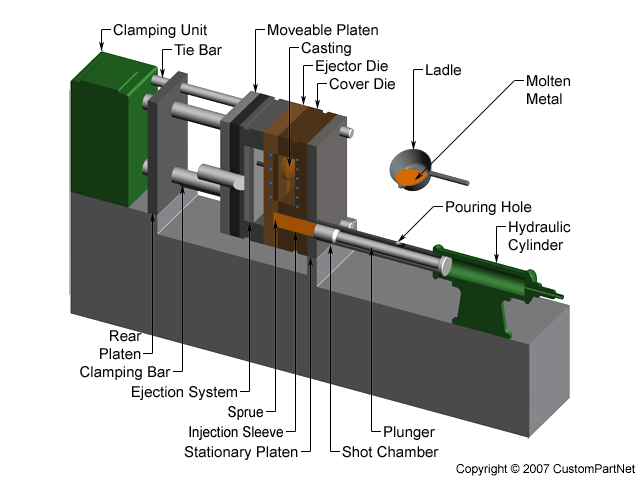This image is a detailed 3D rendering of metal casting equipment, copyright 2007 by Custom Part Net. The model, predominantly dark gray with forest green sections, showcases various components essential for the metal casting process. Suspended above the machine is a cast iron ladle filled with molten metal, labeled accordingly. The machine is divided into several sections, starting from the left with a clamping unit featuring tie bars that extend to the rear platen. Connected to the rear platen is the clamping bar and the ejection system. The equipment also includes a movable platen leading into the casting area, detailed with ejector and cover dies. Key components such as the sprue, injection sleeve, stationary platen, shot chamber, and plunger are clearly marked. The hydraulic cylinder and pouring hole highlight the molten metal's entry point from the ladle into the machine. The comprehensive labels and color distinctions provide a precise overview of the casting process and machinery structure.